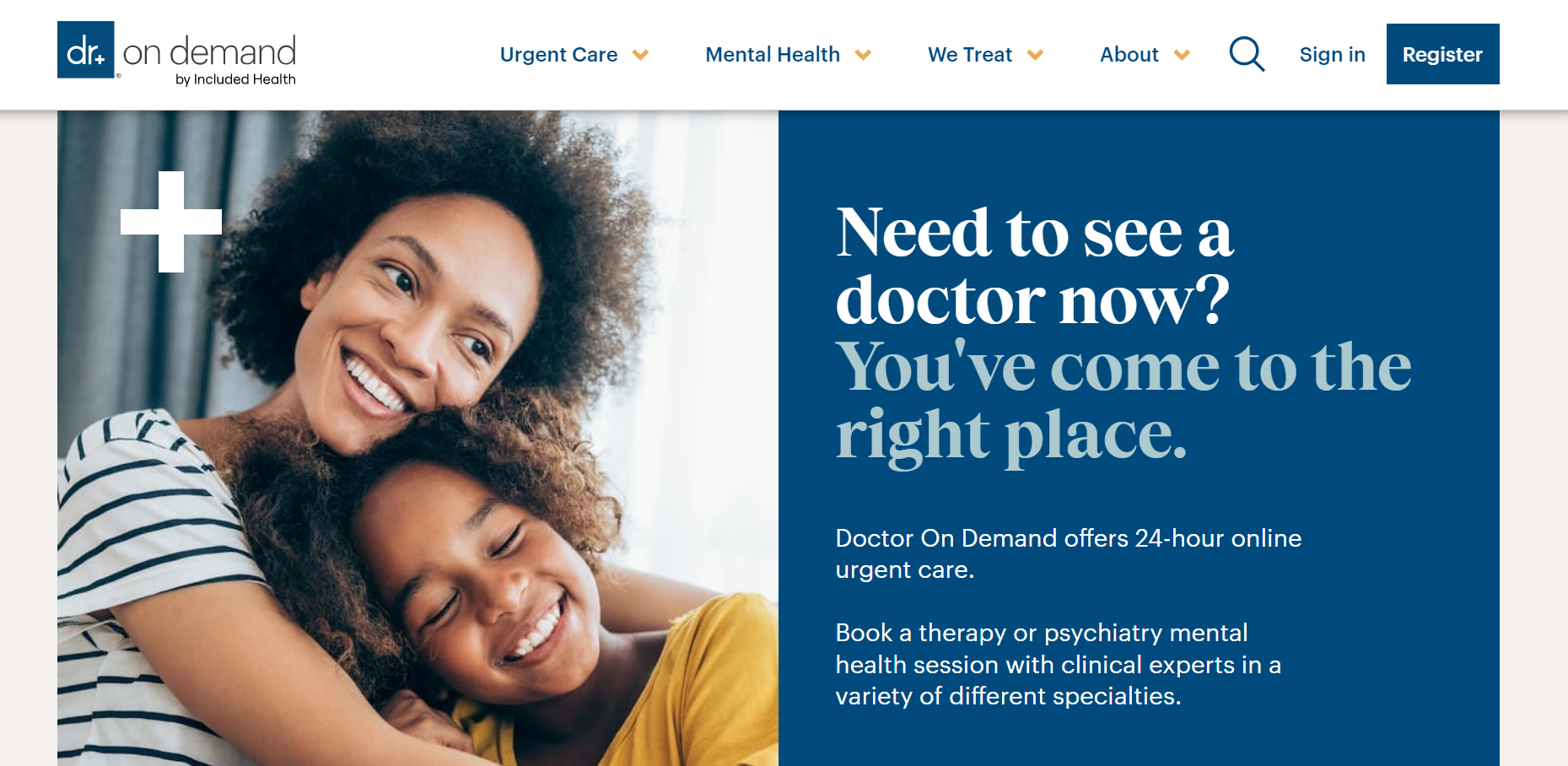The screenshot depicts the homepage of the Doctor on Demand website, prominently featuring a white header with various functional elements. In the header, set against a duo-tone of white and blue, the "Doctor" text appears within a small blue box, while "On Demand" extends into a longer white box. 

Just below, a series of navigation options include "Urgent Care," "Mental Health," "We Treat," and "About," each accompanied by gold-colored drop-down arrows. To the far right, there are options for "Search," "Sign In," and "Register."

Centrally featured is a heartwarming image of a smiling mother lovingly hugging her young child under her chin, both radiating warmth and happiness. In the upper left corner of this image is a subtle plus sign (+).

To the right of this image, a bold blue box contains the text: "Need to see a doctor now? You've come to the right place." Directly below, in white lettering, it explains further: "Doctor On Demand offers 24-hour online urgent care. Book a therapy or psychiatry mental health session with clinical experts in a variety of different specialties." The text emphasizes the convenience and accessibility of both urgent and mental health care services available through the platform.